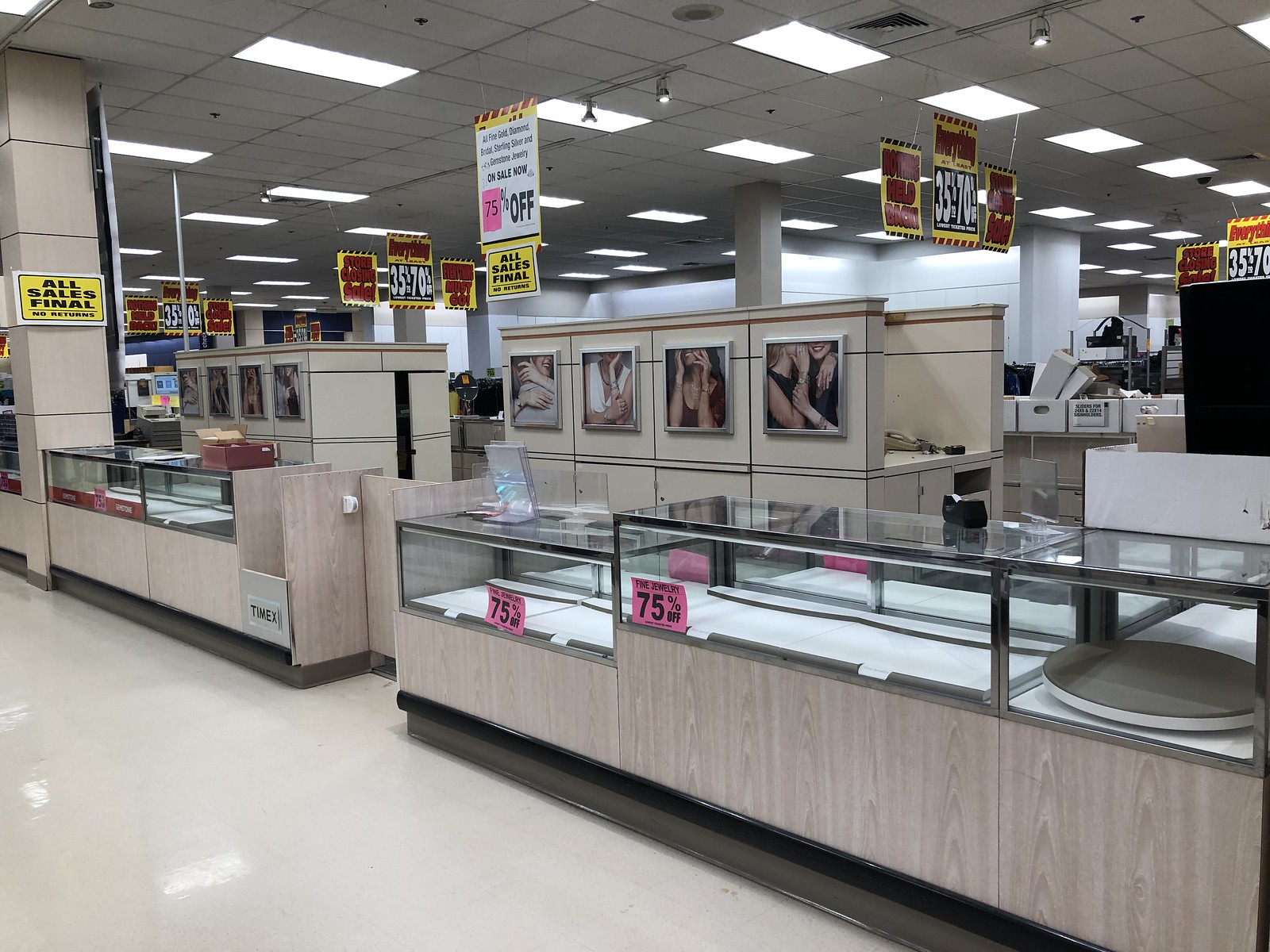The image depicts the interior of a department store, reminiscent of establishments like TJ Maxx or Ross, amidst what appears to be a going-out-of-business sale. The focal point of the image is the jewelry counter, showcased by multiple glass display cases that are completely empty, signaling that the store has likely sold all of its jewelry and watches. Above the counters, bold yellow and black signs declare "All Sales Final, No Returns." Additionally, there are conspicuous pink signs affixed to the cases offering a substantial 75% discount. In the background, more signage is visible, indicating store-wide discounts ranging from 35% to 70% off. Beyond the jewelry counter, various sections of the store such as shoe racks and clothing areas can be seen, similarly marked down. Notably, a Timex sign is attached to one of the boards beneath the jewelry counter, suggesting that the now-empty cases once displayed watches in addition to jewelry.